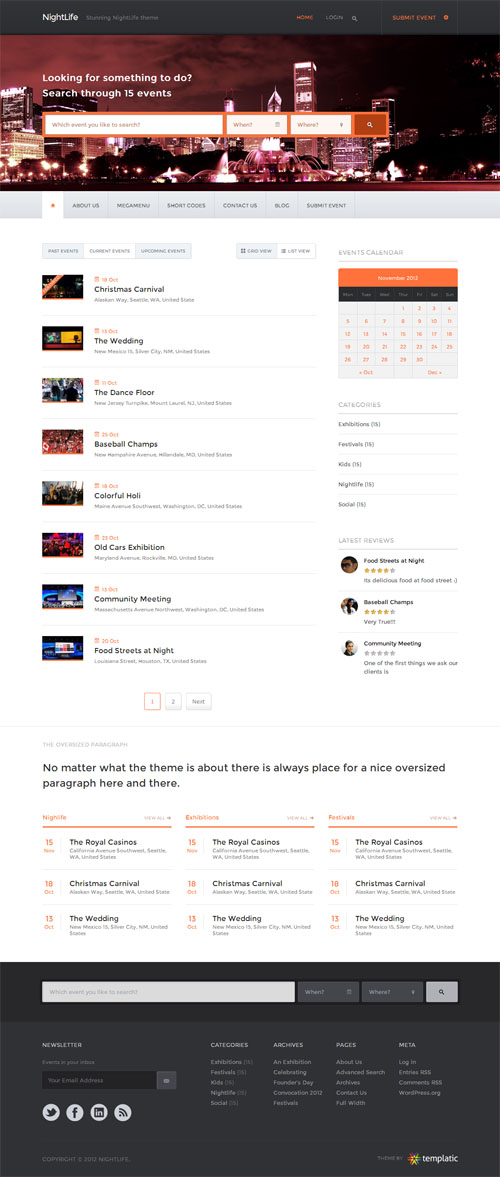This is a blurry, full-page screenshot of a web page, showing both the header and footer in a minimized, flat layout without any need for scrolling. 

### Header:
- **Background**: Nighttime city skyline with illuminated buildings and city lights.
- **Central Text Box**: Prominently positioned.
- **Right Side**:
  - **Two Drop-Down Boxes**.
  - **Search Bar**: Includes a magnifying glass icon for searching.

### Body:
- **Background**: White.
- **Left Side**: Vertical arrangement of thumbnails.
- **Right Side**:
  - **Titles**: Bold black font.
  - **Information**: Light gray font directly beneath titles.
  
### Sidebar:
- **Top Right**: Small calendar with a gray background, featuring orange and black bars above it.

### Footer:
- **Components**:
  - **Search Bar**: Gray.
  - **Two Drop-Down Boxes**: Dark gray.
  - **Social Media Logos**: Located at the bottom left, featuring Twitter, Facebook, Instagram, and LinkedIn icons.

The overall image is out of focus, making the details difficult to discern, but the general layout and structure of the web page are evident.